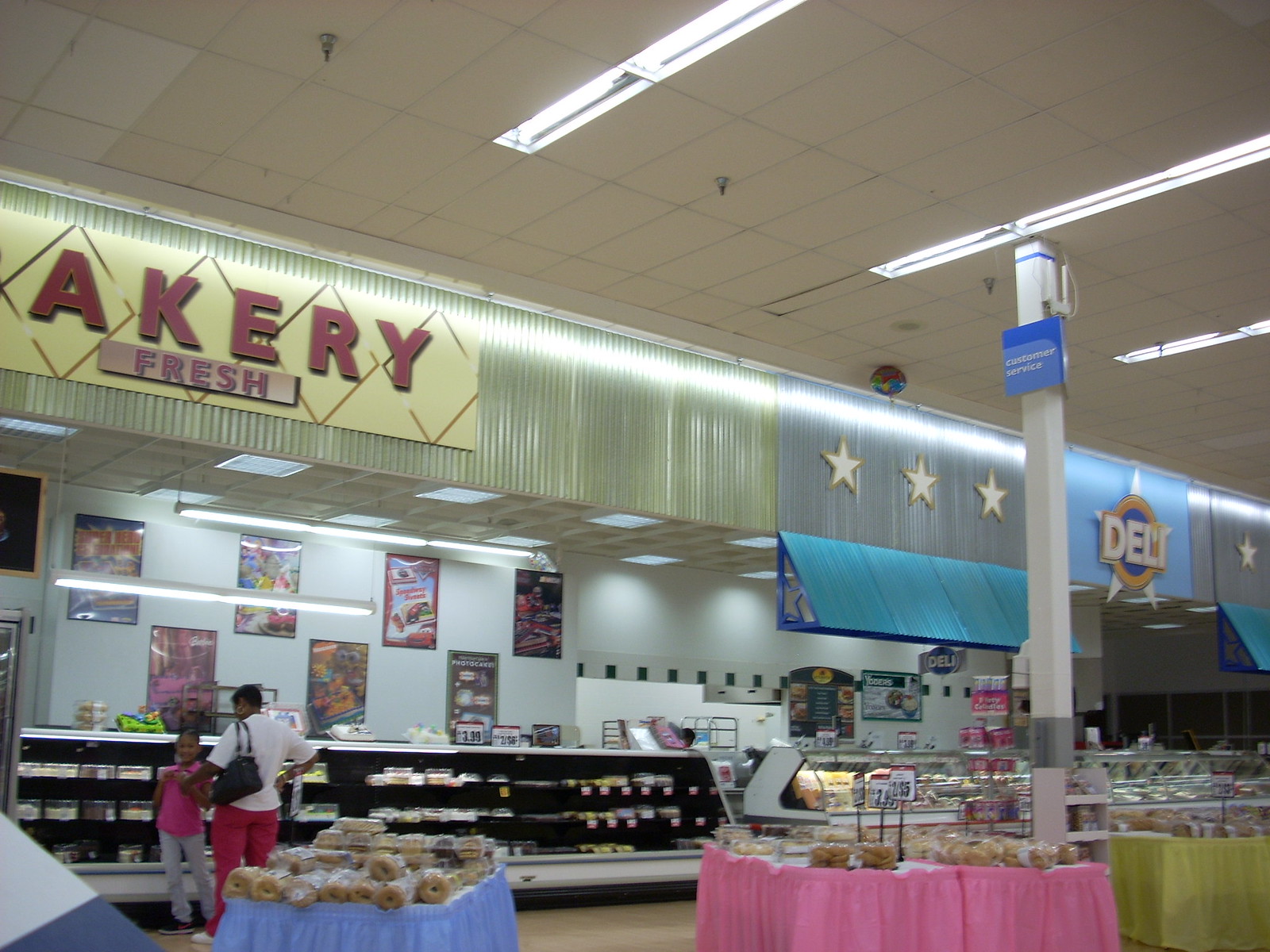The photo captures an interior view of a grocery store, focusing on the bakery and deli sections. In the foreground, there's a bustling bakery area on the left with shelves stocked with an array of cakes and other treats. To the right of the bakery lies the deli counter, featuring a clear display case showcasing a variety of meats. A mother and child are seen at the bakery, waiting to be assisted. Front and center in the image, there are several tables adorned with vibrant tablecloths in pink, blue, and green, each table displaying different items available for purchase. The scene is lively and inviting, suggesting a well-organized and customer-friendly environment.